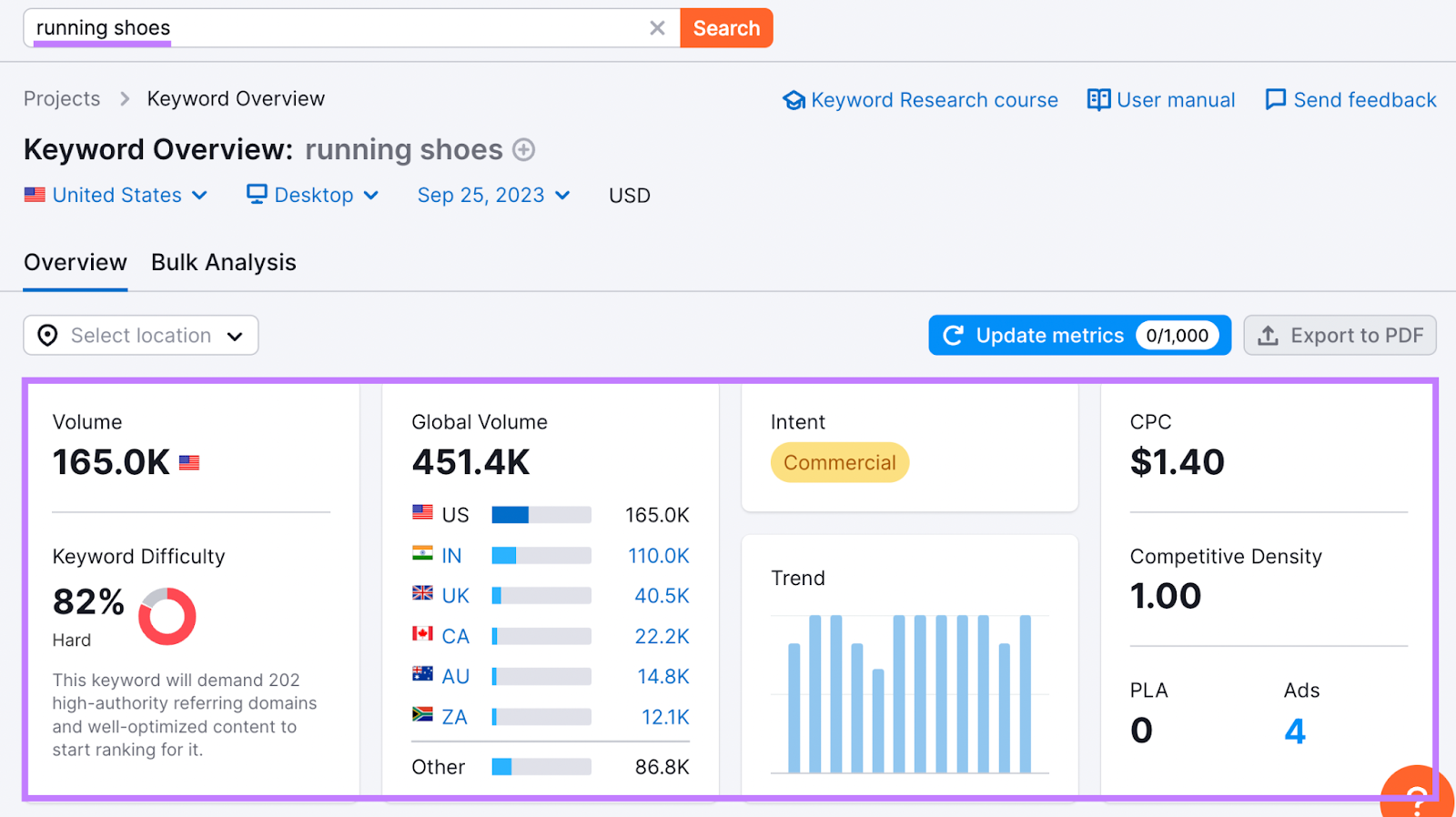This image is a screenshot of a price index, specifically focusing on keyword metrics for "running shoes". Located at the top left corner, next to the search box, is the text "running shoes." Below this, the image displays sections labeled "Projects," "Keyword Overview," and "Keyword Overview Running Shoes United States Desktop September 25th, 2023 USD."

Key metrics featured in the screenshot include:
- Volume: 165.0K
- Keyword Difficulty: 82% (Hard)
- Global Volume: 451.4K
- CPC (Cost Per Click): $1.40
- Competitive Intensity: 1.00